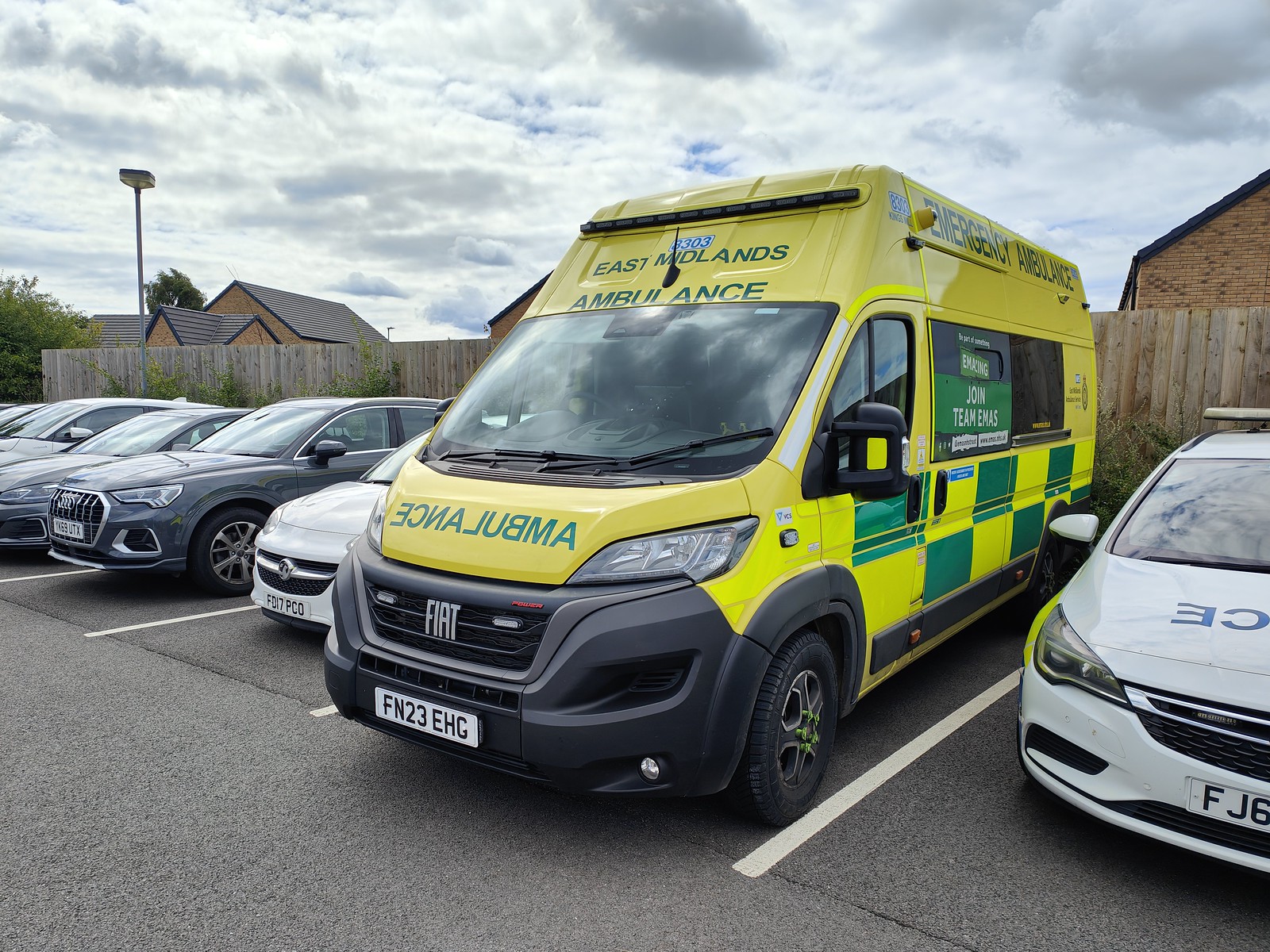The photograph, taken outdoors on a cloudy day with white and grey clouds and glimpses of blue sky, prominently features a yellow Fiat ambulance. The text "East Midlands Ambulance 8303" is written in green on the sides, along with alternating yellow and green panels at the bottom. The side doors bear a call to action with phrases like "Join Team EMAS" and social media handles, while the license plate reads FN23EHG. The ambulance is parked in a lot marked with white lines, surrounded by various sedans including a white police car with the words "CE" on its bonnet. In the background, wooden fences enclose rooftops of houses, interspersed with small plants, trees, and lampposts.